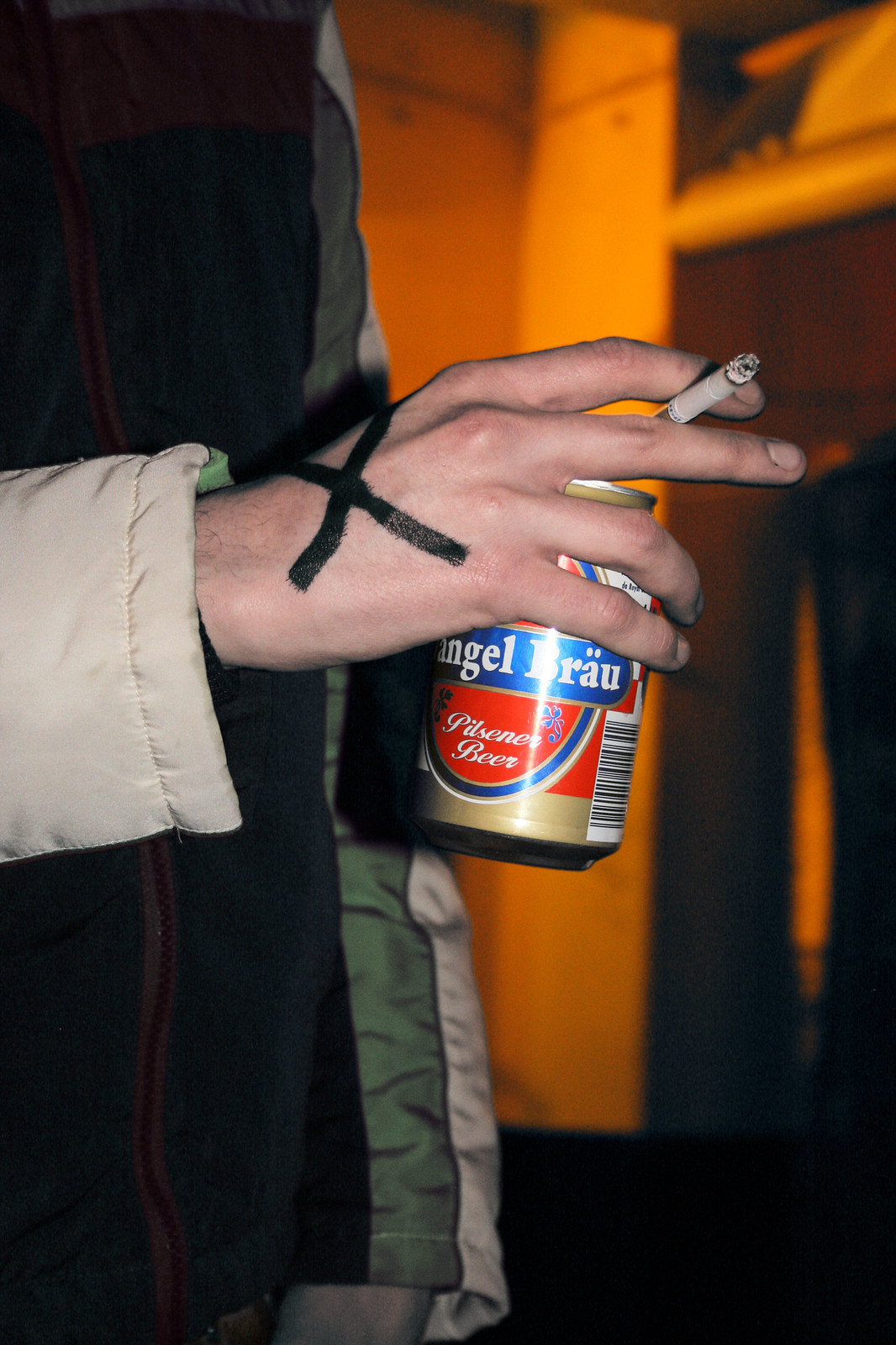The image captures a close-up of a Caucasian person’s right hand and torso at an indoor setting, likely a party. The individual is holding a lit cigarette, with ash at the tip, between their fingers, and beneath it, they grip a can of Pilsen beer. The beer can features a blue and red label with white writing, and the top and bottom are gold-colored. A prominent black X is painted on the back of their hand. The person's attire is distinctive, with an old-fashioned jacket showcasing a tan sleeve with green trim, and the body of the jacket appears to mix green, cream, and black fabrics. The background, while dimly lit, reveals tan-colored cabinets and what appears to be a curtain rod with clothes hanging on it, suggesting a domestic setting. The picture is taken from a very close angle, making it tough to see the person’s face or much else beyond these details.